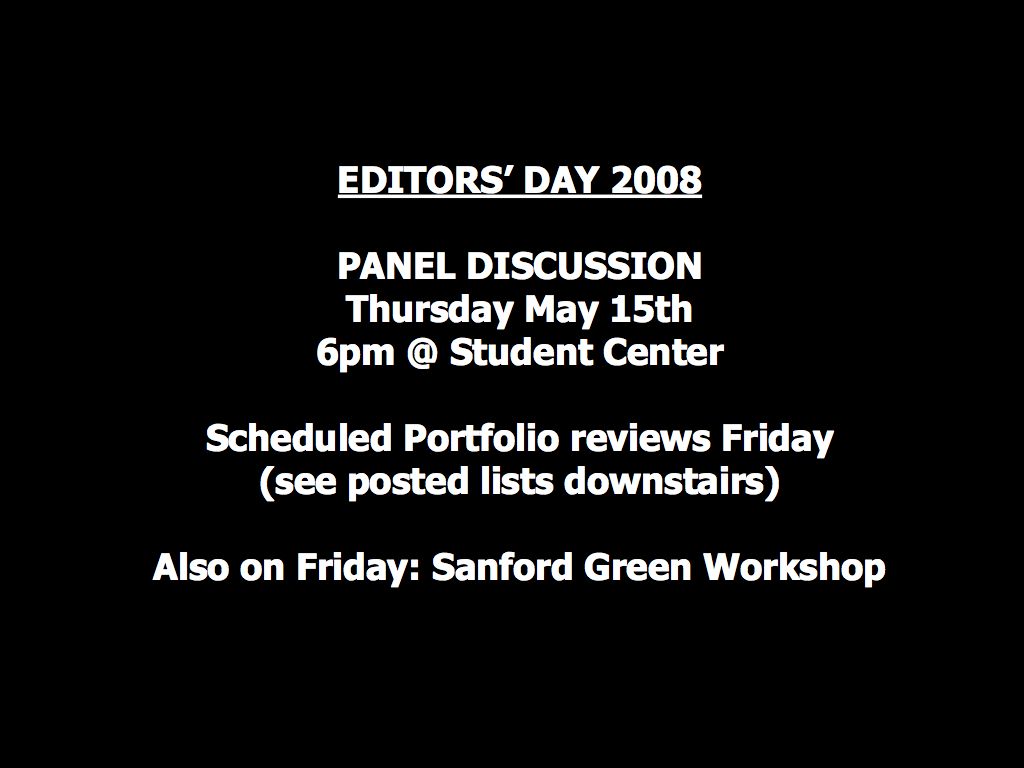The image features a clean black background with centered white text in a medium font, all highlighting key event details. At the top, in all capital letters, underlined, it reads "EDITORS' DAY 2008." Below this, the event details follow in a non-caps format: "Panel Discussion," "Thursday, May 15th," "6 p.m. at Student Center." Further down, it continues with "Scheduled Portfolio Reviews Friday," and in parentheses, "see posted list downstairs." The final line notes, "Also on Friday, Sanford Green Workshop." The entire text is uniformly spaced and arranged on a horizontal, rectangular background, providing clear, important event information.